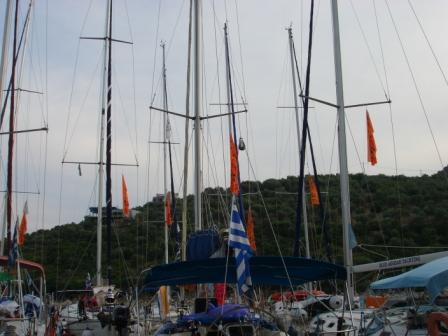In this image, a cluster of sailboats dominates the scene, their tall masts crisscrossed with ropes reminiscent of a ship's rigging. Each mast prominently displays an orange flag, and a partially unfurled Greek flag is seen front and center. The boats, varying in colors including dark blue, light blue, orange, and red, are mostly visible through their towering sails, with only a few glimpses of their hulls at the bottom. Behind the boats, a green hill with trees and bushes rises under a sky that shifts from a pale blue on the left to a more grayish hue on the right. The bottom features a mix of indistinct shapes, including a light blue form on the lower right-hand side that appears to be a boat cover or tent. The overall backdrop is calm yet bustling with the activity of a port or docking area.